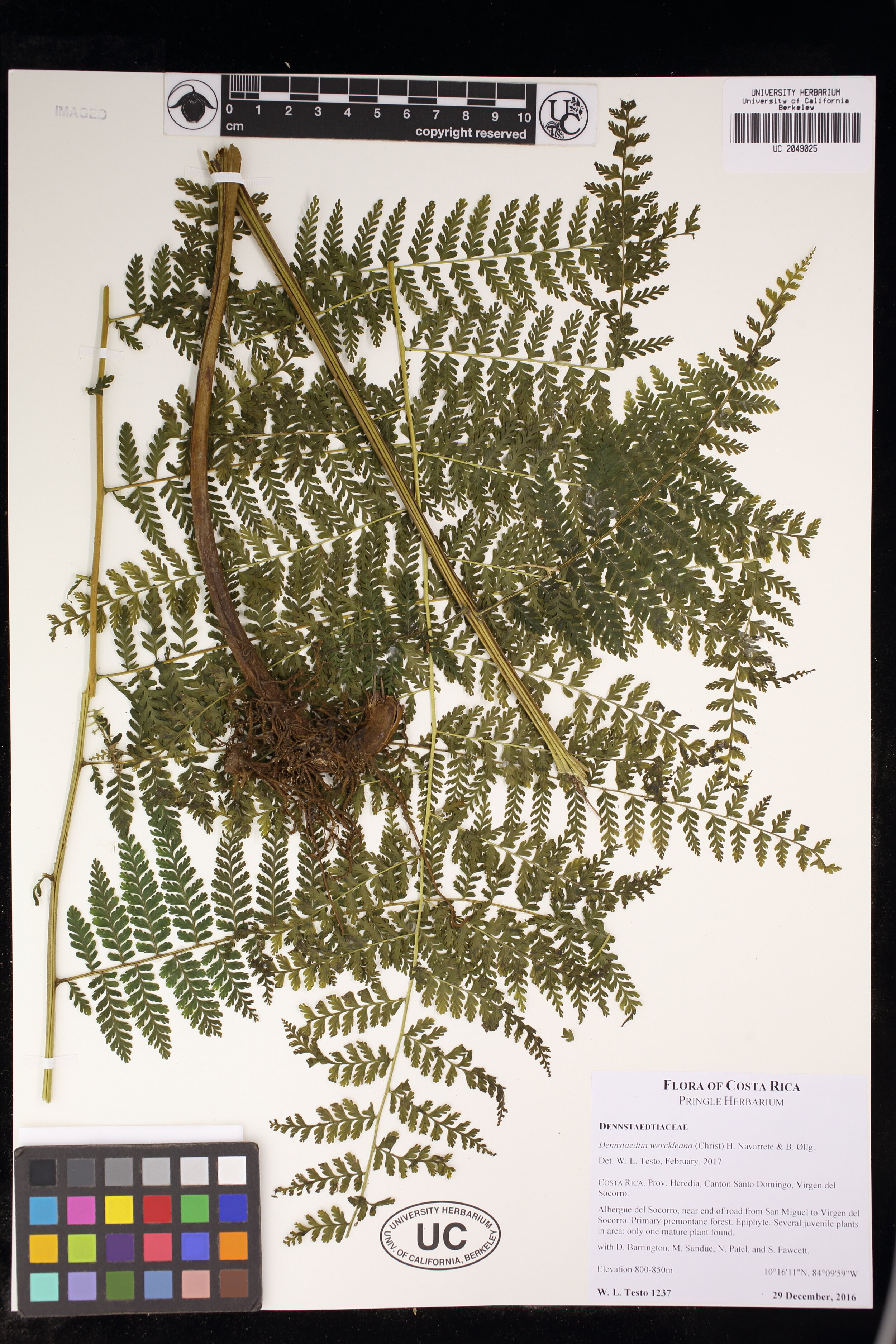This poster displays a comprehensive array of green fern leaves, meticulously arranged for identification purposes. The ferns are spread across a white background, showcasing numerous branches, each with intricately crossing leaflets. The entire image is framed by a black border, with a prominent black bar at the top featuring indecipherable white icons. Adjacent to this bar is a ruler scale in inches, ranging from zero to ten, aiding precise measurement. The upper right corner hosts a barcode and label, while the bottom left corner is adorned with a detailed palette of color squares in various shades—from black and gray to vibrant hues of blue, pink, yellow, and more. A distinctive oval with the letters "UC" in black lettering sits prominently at the bottom center of the poster. Along the right side, a header and subheader—announcing the "Flora of Costa Rica"—are accompanied by a detailed description in small print, too fine to be legible from the image. This detailed poster serves as an essential tool for identifying different fern species.